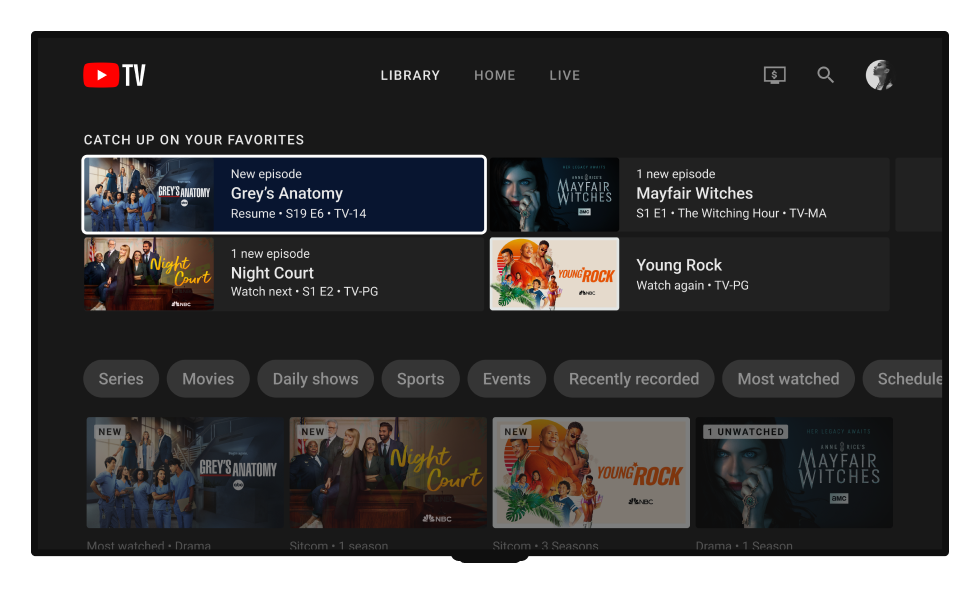The image displays a web page with a layout reminiscent of a TV guide, featuring a sleek black background. Dominating the upper section is a red YouTube logo with a white triangle pointing right, paired with the text "TV" in bold white font centrally placed. Smaller white fonts spell out "Library," "Home," and "Live" in the middle section of the header.

To the right, a cluster of icons is visible, including a small monitor screen with an "S" in the center and a magnifying glass emblem – presumably a search function. Nearby, there is a round profile image with a white background showing the side profile of a person.

Below this header, the primary content is arranged in sections. Starting from the top left, there is a white box with the prompt "Catch up on your favorites." Below it, the heading "New" highlights popular shows like "Grey's Anatomy." There's a thumbnail featuring the cast in blue scrubs next to text reading, "Resume S19E6 - TV14."

To the right, another show, "Mayfair Witches," is showcased. The image depicts a woman with her hands near her eyes. Accompanying text indicates, "One new episode: Mayfair Witches S1E1, The Witching Hour, TV-MA."

Continuing rightward, "Night Court" is promoted with an image of the cast and the iconic yellow logo. Text proudly announces, "One new episode: Night Court - Watch Nest S1E2, TV-PG."

Lastly, to the extreme right, "Young Rock" is featured, likely referencing Dwayne Johnson's TV show. An orange circle backdrops the cast image, with the text beneath stating, "Young Rock - Watch Again, TV-PG."

Underneath this, a series of grey circular icons offers various categories: "Series," "Movies," "Daily Shows," "Sports Events," "Recently Recorded," "Most Watched," and "Schedule."

At the bottom, the same four show images are repeated, although they appear more faded, with some additional white text below them, which remains somewhat indistinct.